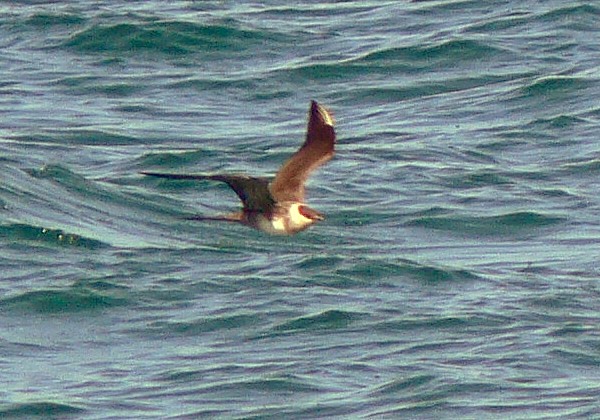This rectangular color photograph, approximately four inches high by five inches wide, captures a vibrant outdoor scene during the daytime. The grainy and somewhat blurry image presents the ocean with blue-gray to dark green waves and visible water turbulence. In the center of the composition, a seagull-like bird with a slender, light tan to white underbelly and brown wings is the focal point. The bird's large, pointed beak and slightly pointed head are prominent as it flies from left to right above the water, which appears disturbed beneath it. One wing extends above the water's surface, contributing to the overall dynamic feel of the image. The bird's body may seem a bit compressed, as if it had recently touched the water. The photograph, which has a nostalgic quality reminiscent of older times, emphasizes representational realism despite its imperfections, capturing the natural essence and subtle motion of the scene.